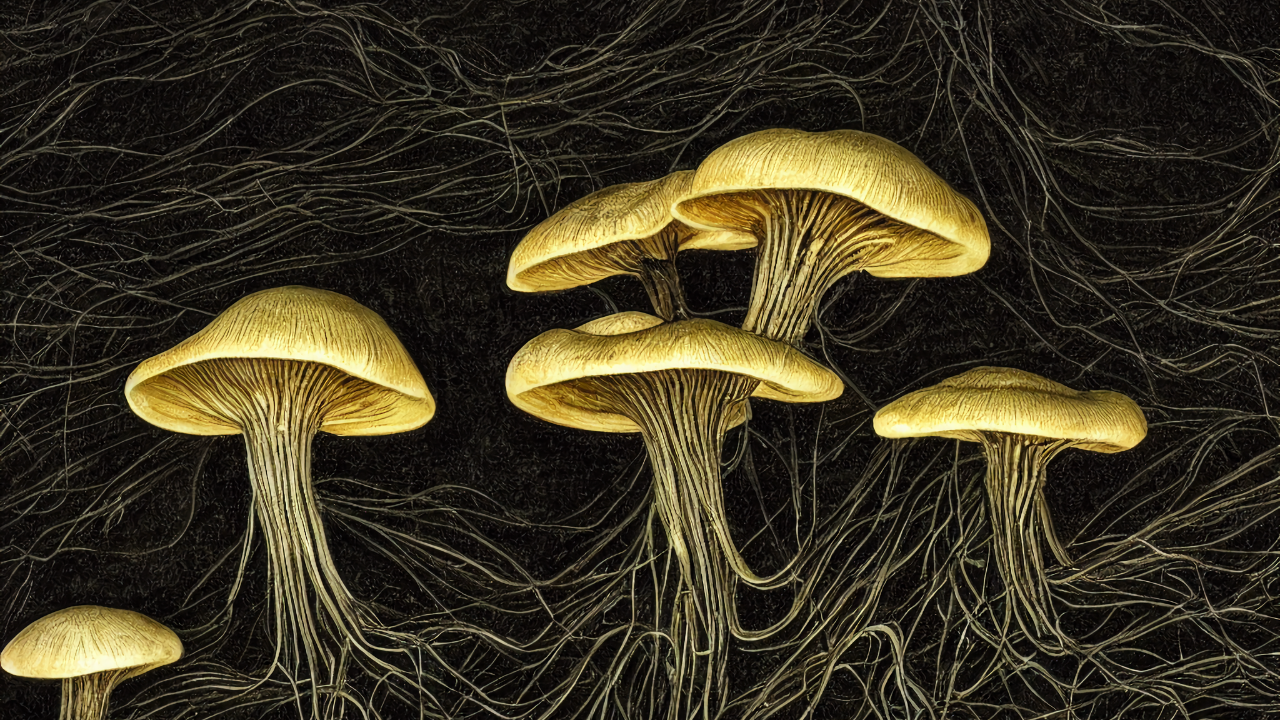This horizontally aligned rectangular image features a dark, cobalt background sprinkled with tiny gold and white specks that resemble stars, creating a night-sky-like effect. Dominating the image are six organisms that could be interpreted as either mushrooms or jellyfish due to their shared characteristics. These organisms, depicted in shades of gold and tan, have rounded tops similar to the hoods of jellyfish or mushroom caps. From their undersides, numerous hair-like strands or tentacles unfurl, some intertwining and others floating freely, adding to the sense of ethereal movement. The largest organisms are situated in the middle right, while the smallest can be found in the lower left and right corners. Each organism is intricately detailed with thin black lines extending downwards, enhancing the delicate and intricate nature of these fascinating entities.